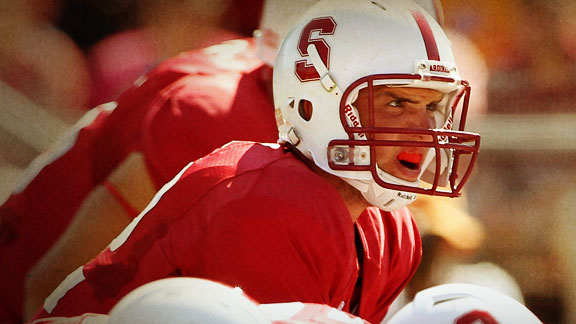This close-up photograph captures a football player in the heat of the game, with the dominant colors being red and white. He is wearing a red jersey with a white number on the back, and a white helmet featuring a red "S" on the side along with a red stripe on the crown. His helmet also includes a red faceguard. The player's face is scrunched into a scowl, his mouth open to reveal a red mouth guard protecting his upper teeth. The image focuses primarily on his upper body, showcasing his red and white uniform and intense expression. In the background, just behind him, there's a glimpse of another player dressed similarly, with only part of his helmet and his tan arm, adorned with a red arm band, visible. The backdrop is a blurred mix of indistinguishable shapes and colors, with hints of red, beige, white, and a touch of purple, emphasizing the foreground action and the player's concentrated demeanor.